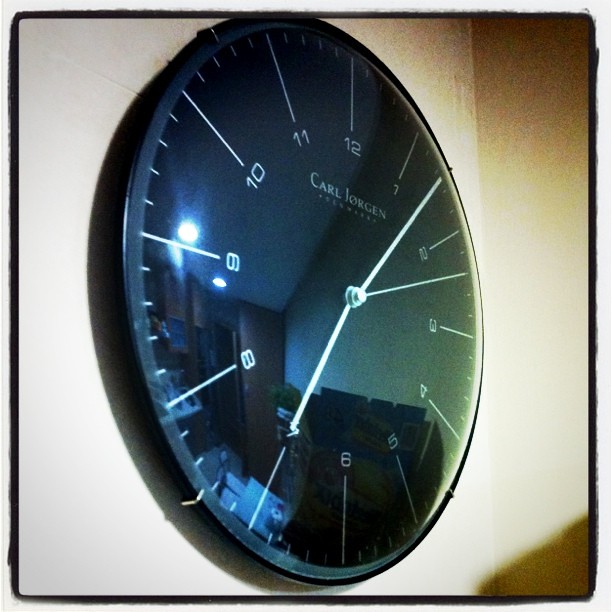This color close-up photograph, taken at a 45-degree angle from the left side, captures a round wall clock with a black frame and a sleek black face. The clock is secured on a cream-colored wall that appears grainy, with shadows in the bottom right and top right corners. The clock's white hour and minute hands are positioned to show the time as 7:07, with the hour hand just above the 7 and the minute hand between the 1 and the 2, while the second hand is between the 2 and the 3. The clock face features prominent white numbers and thick lines marking each hour, with thinner white lines for the minute indicators. Below the 12 o'clock position, the branding text reads "Carl J-Ø-R-G-E-N," with a distinctive line through the "Ø." The clock is encased in a glass or plastic dome, which reflects the room's ambient elements, including a faint outline of a door and a light glare near the 9 o'clock position, adding depth to the image.